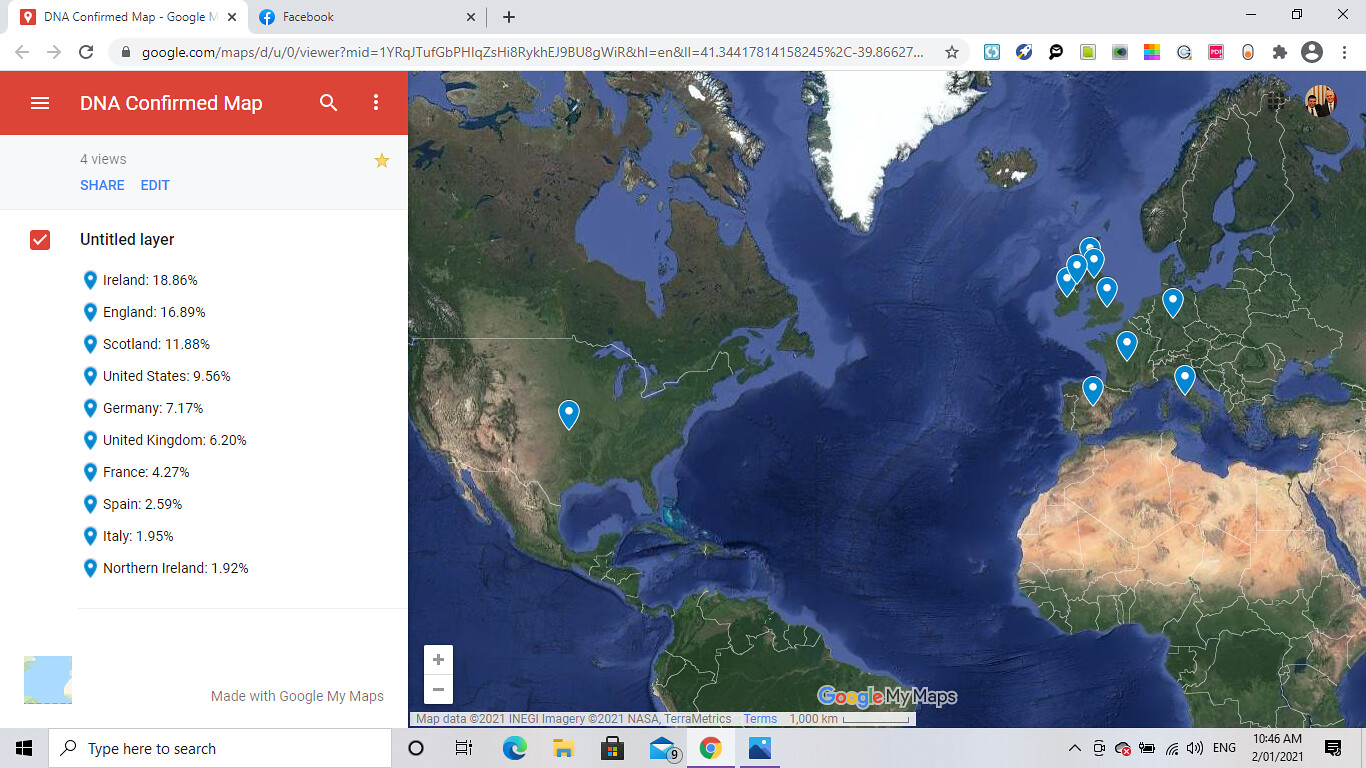Here's a polished and highly detailed caption for the image described:

"The image is a wide screenshot of an open browser window displaying DNA mapping results. At the top of the browser, the leftmost tab features a red logo, accompanied by partially visible text that reads 'DNA confirmed map-googlem,' suggesting it may be related to Google Maps. The adjacent tab, which is gray and inactive, shows the Facebook logo. Below the tabs, an orange box prominently displays 'DNA confirmed map,' followed by a gray box indicating 'four views,' with options in blue font labeled 'share' and 'edit.' A yellow star icon is positioned on the far right of this section. Further down, there's a section labeled 'untitled layer,' detailing percentages of DNA origins: Ireland 18.86%, England 16.89%, and other European countries, with the exception of the United States. The right-hand side of the screen features a large world map with clearly marked borders, although country names are not specified. Blue arrows on the map point to various regions, corresponding to the data points listed in the table on the left."